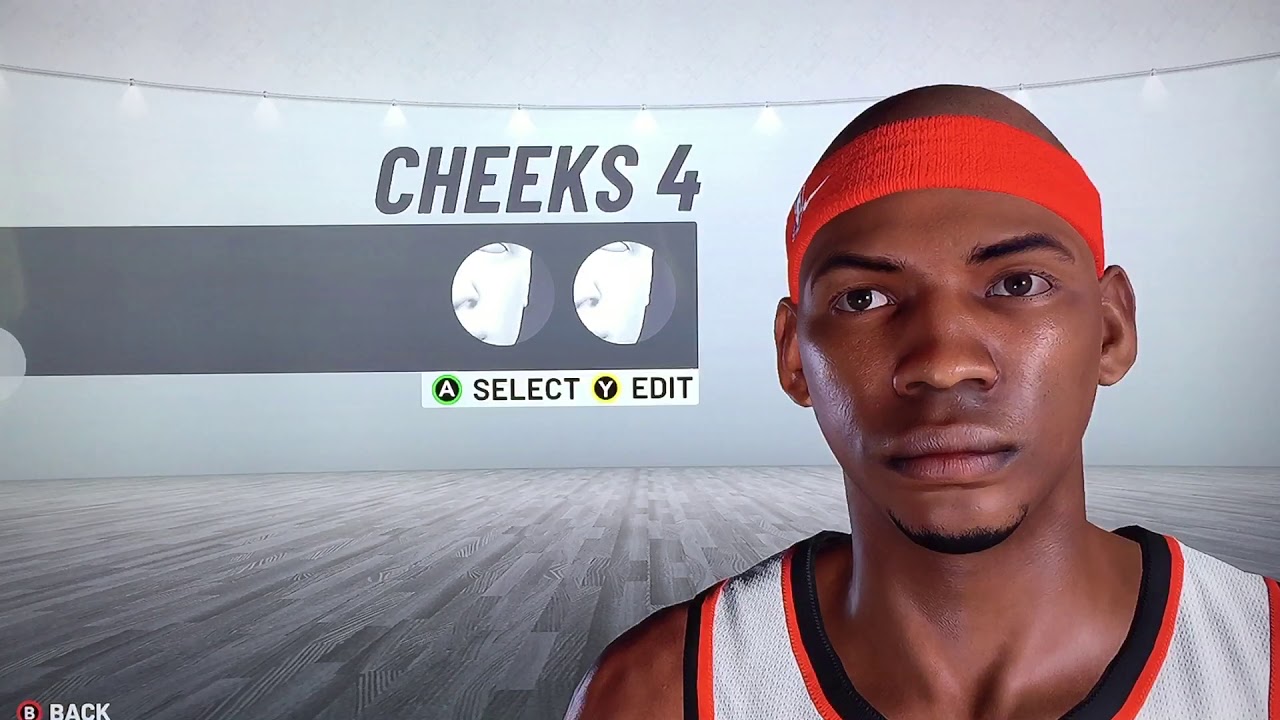This image is a detailed digital screenshot from a video game. 

In the bottom left corner, the interface shows navigation options with "B" in a circle labeled "Back," an "A" in a green circle labeled "Select," and a "Y" in a yellow circle labeled "Edit." 

Dominating the right side of the image is a digital drawing of a basketball player. The character is a dark-skinned male with distinctive features, including a black goatee and eyebrows. He is bald but wears a green sweatband with a small emblem on the left side, positioned over his eyebrows. His eyes are visible, and he appears to be looking slightly to his right. 

The player is dressed in a white short-sleeved basketball jersey adorned with orange and black stripes. Detailed rendering includes visible veins around his neck, but there is a notable absence of an Adam's apple. Both of his ears are visible, though the image does not reveal the back of his head or body.

In the center of the screen, the word "Cheeks" is displayed in gray text, with "C-H-E-E-K-S" spelled out and a number "4" beneath it, underlined by a thin gray stripe with circular accents. The background features a gray color, highlighted by a sweeping pattern that might resemble a stylized basketball court but lacks any actual depictions of a basketball or court. This setting suggests an indoor gymnasium atmosphere.